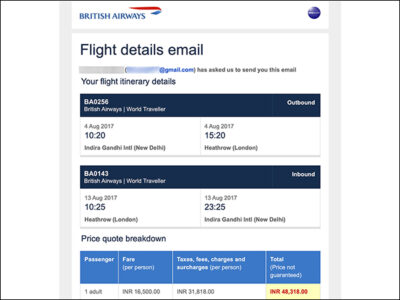In the image for a flying service, the top left features the name **British Airways** in blue text, accompanied by the British Airways logo—a blue and red ribbon-like design—positioned to the top right of the name. To the extreme top right corner, a purple circle contains white text. Centered towards the top, slightly to the left, the words "Flight Details Email" appear in black lettering, with a blurred email address beneath for privacy protection. Below this, the phrase "Your Flight Itinerary Details" is displayed, followed by a boxed section. Within the top left corner of this box, **"BA0256"** is listed, with "British Airways World Transfer" below it.

Proceeding further down, two white boxes sit side by side. The left box has the date and time **August 4th, 2017, 10:20**, while the right box reads **August 4th, 2017, 15:20**. Below this section, another flight number, **"BA0143"**, is noted, leading to two additional white boxes. The left one states the details **August 13th, 2017, 10:25**, and the right one notes **August 13th, 2017, 23:25**.